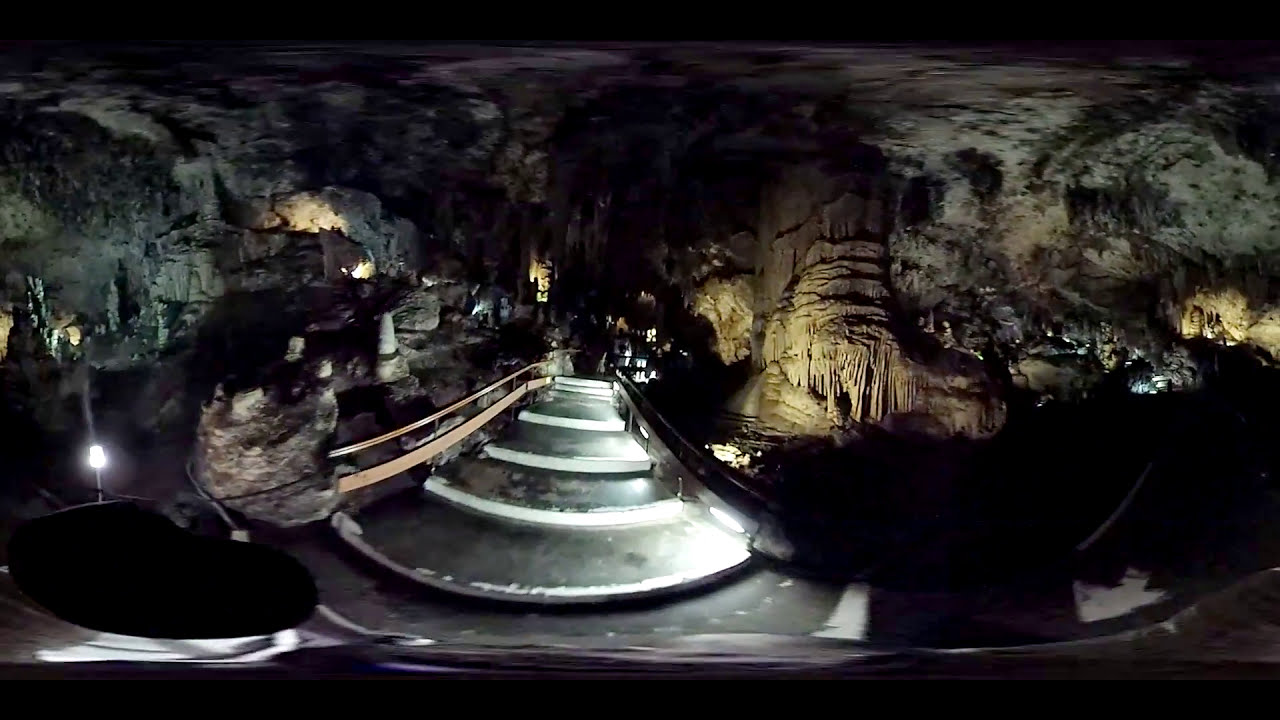The horizontal rectangular image is shrouded in darkness, making the scene somewhat ambiguous at first glance. Dominating the center of the image are rounded steps with white edges, transitioning into gray concrete, leading upwards. These steps are framed by railings on either side. The right side of the image reveals a large brown stone building with bushes and a tree in front of it, and some lights glow faintly from within. On the left, there's a suggestion of houses or another type of building, similarly lit. Between these buildings, the steps ascend, their reflective surfaces capturing ambient light from various sources. The overall scene conjures an eerie atmosphere, reminiscent of an old urban setting or possibly even a cave with dark, green rocks, adding to the mystique with their wet, glistening surfaces.